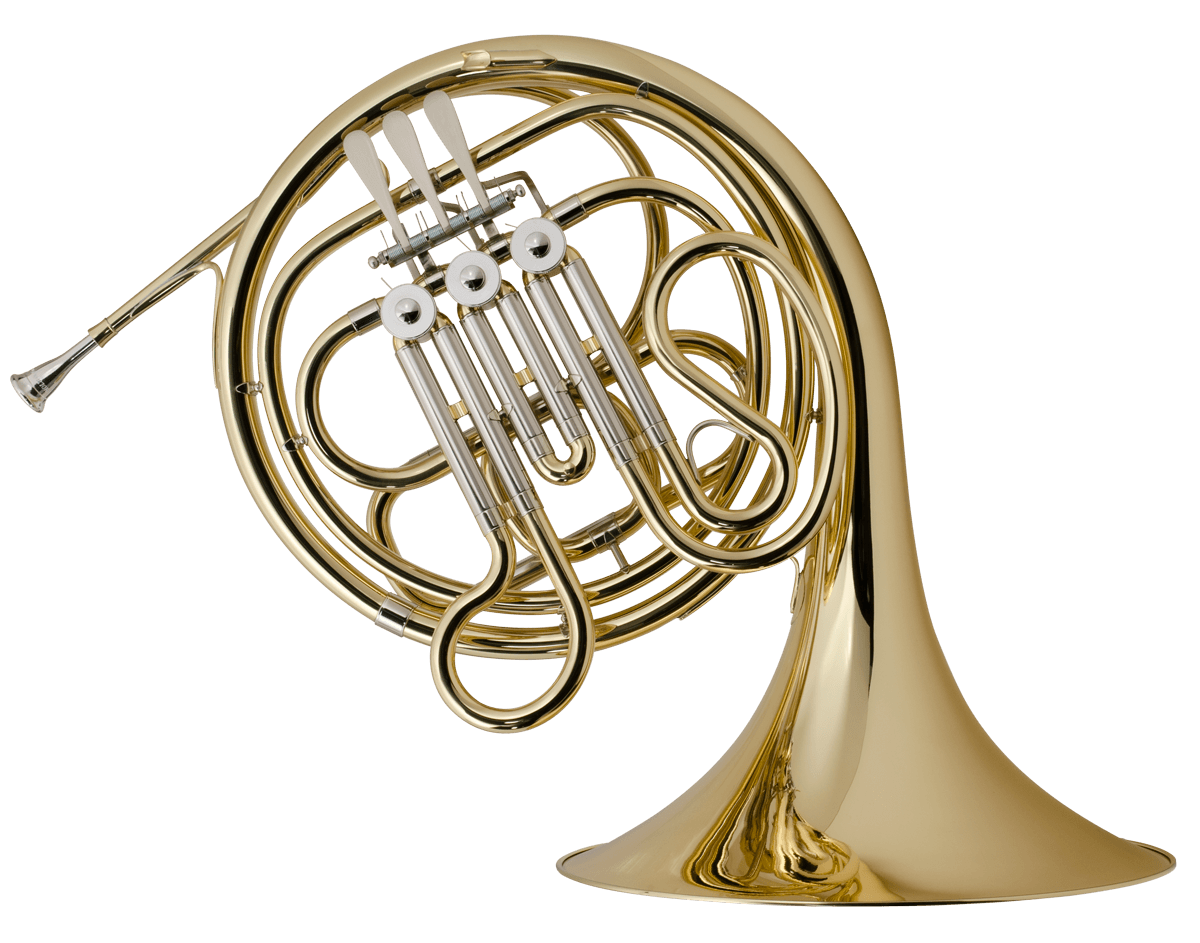The image depicts a beautifully intricate French horn prominently displayed against a pristine white background. The instrument is primarily a light, shiny gold, adorned with numerous swirly circles that create a sense of complexity akin to a giant jigsaw puzzle. The mouthpiece, situated on the left side, stands out in silver, contrasting elegantly with the gold body. The horn's intricate tubing interweaves through the design, with some sections accented in silver, particularly where the tubes extend into the larger bell. Three silver-tinted finger valves, almost whitish in color, are centrally located, accompanied by silver screws. The horn is notably reflective, capturing the light and reflecting parts of its own structure, particularly where the middle tubes intersect. This French horn, with its ornate and meticulously crafted design, not only stands out as a functional musical instrument but also as a potential art piece.